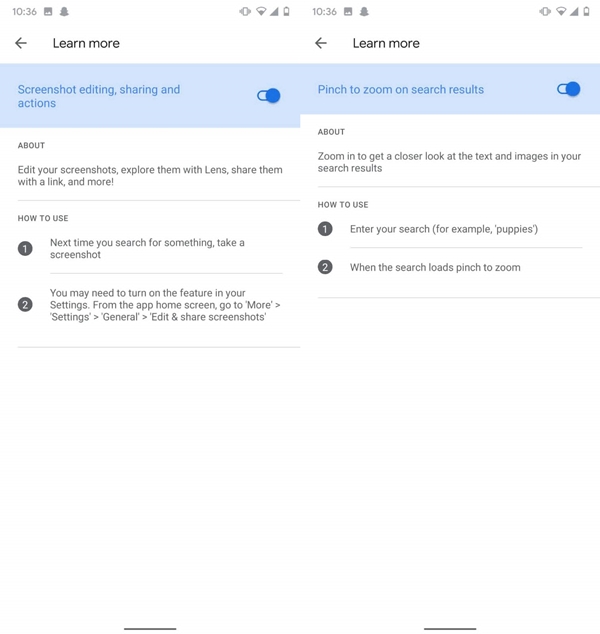The image displays a split-screen view, captured on a smartphone, showcasing instructional guides for two different features. Both screens at the top display identical status bars with the time "10:36," along with icons for signal strength, Wi-Fi, and battery life. 

Each screen includes a title at the top, a "Learn More" link, and a directional left arrow. Below the arrows, a blue-highlighted slider button is positioned to the right, indicating that the views are aligned.

On the left screen, the heading reads "Screenshot Editing & Sharing Actions," highlighted in blue. Below this, the section labeled "About" describes the features: "Edit your screenshots, explore them with lenses, share them, and link them." Instructions under "How to Use" state: 
1. "Next time, search for something like a screenshot."
2. "You may need to turn on the feature in settings from the app home."

On the right screen, the heading reads "Pinch to Zoom in on Search Results," and is similarly highlighted in blue. The "About" section explains that users can "Zoom in to get a closer look at your text and image in search results." The "How to Use" instructions state:
1. "Enter your search, for example, puppies."
2. "When the search loads, pinch to zoom."

Both screens use a white background, with light gray numbering for the steps and bolded "Learn More" links. The highlighted areas and the slider button contrast in blue, making the instructions clear and visually distinct.